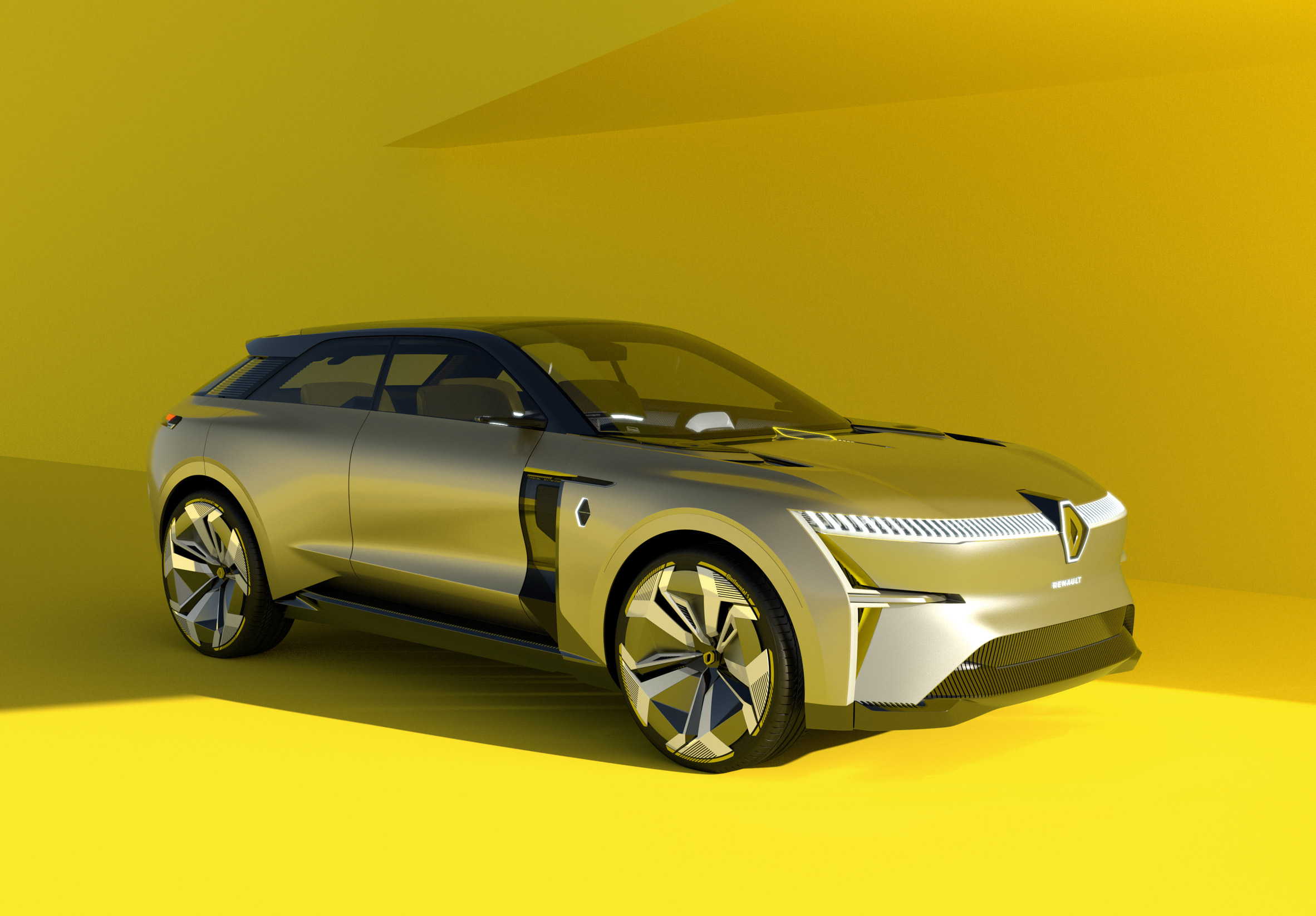In this image, a futuristic, chrome-finished SUV concept car is showcased against a yellow backdrop with shaded areas that emphasize the sleek design of the vehicle. The car, which is depicted in a 3D computer-generated artwork, features large, five-spoked chrome wheels with thin black tire walls and yellow cores between the spokes. It has a distinctive light bar that wraps around the rounded front and extends vertically as small dashed lights over a white panel, flanking a diamond-shaped silver logo in the center of the front grille. The SUV exhibits a curvy, glass roof and windshield, with a black hood air scoop near the passenger door and a black channel running between the tires. The vehicle's body is primarily silver, with a striking modern design that includes unconventional headlight styling and a smooth, aerodynamic profile. The car is a two-door, four-seater model, oriented to the right, capturing the light source that enhances its shiny, chrome exterior.